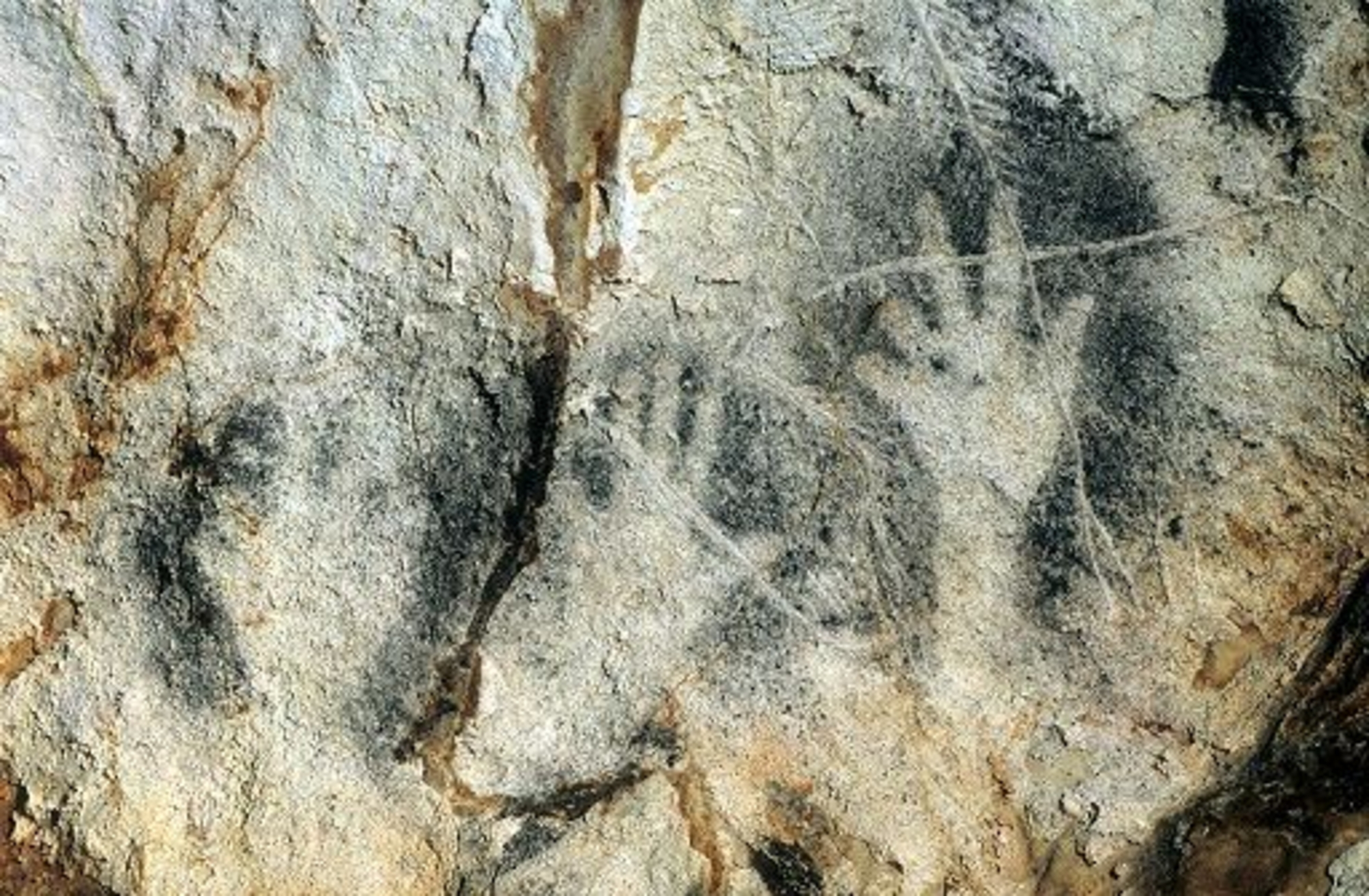This close-up photograph showcases a rock formation with a predominantly grey and brown surface, accented by some rust and copper tones. Prominently featured are three hand imprints, which are the same color as the rock itself, surrounded by areas of black paint, giving the impression that someone placed their hands on the rock and then spray-painted around them. There is also a large crack running through the middle of the rock, adding to the texture and complexity of the surface. The right side of the image is particularly dark, with significant black areas, likely from the spray paint. This image bears a resemblance to ancient cave drawings, creating an intriguing blend of natural and human-made elements.